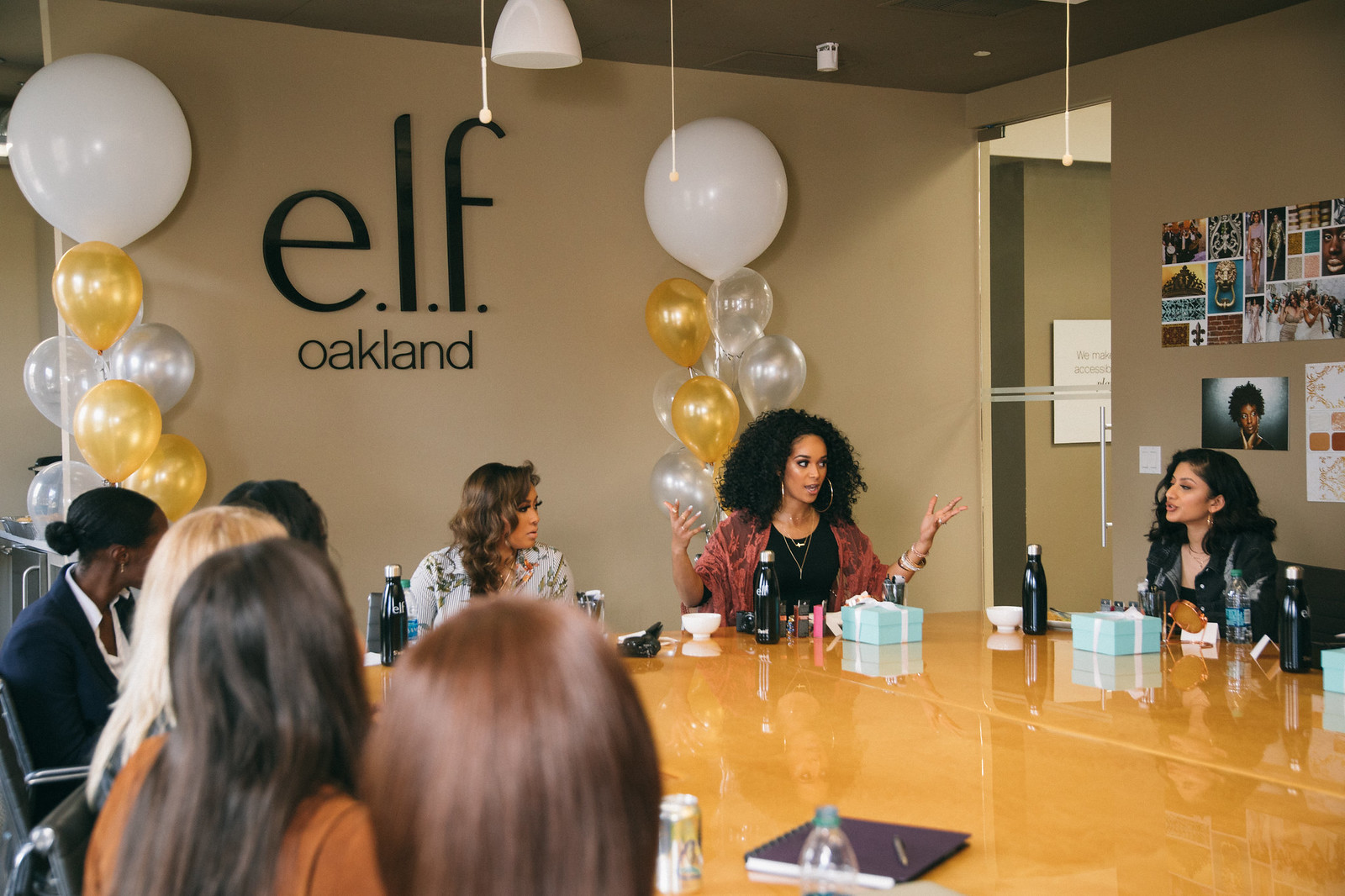In the image, a group of individuals is seated around a tall, glossy, tan-brown table, suggesting a work meeting environment. On the beige wall in the background, the brand name "E.L.F. OAKLAND" is prominently displayed in black lettering. Decorating the space, white, gold, and silver balloons flank the brand name, with the largest balloon being white and positioned at the top center.

Each person visible in the frame has a pastel blue gift box adorned with a white bow in front of them. A woman stands out as she speaks; she has voluminous, curly hair and is dressed in a red sweater over a black shirt. She accessorizes with large hoop earrings and has her eyes heavily outlined with black eyeliner, fitting for a makeup company setting.